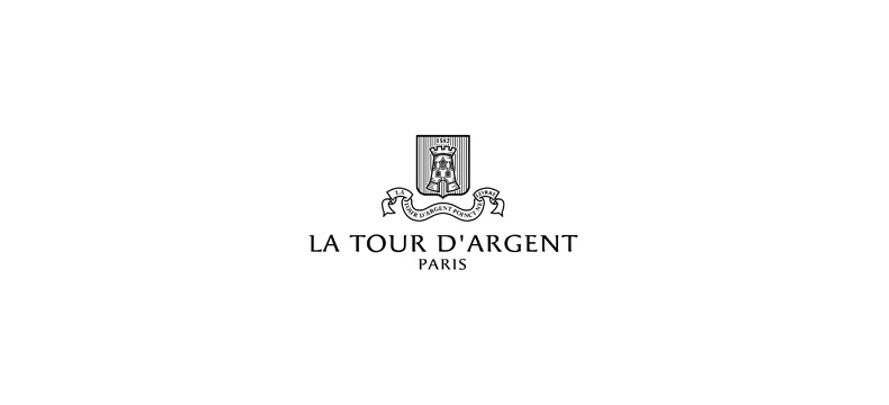On a solid white background, the image showcases a logo and the name of a company, prominently centered. The logo itself is square-shaped, bordered by a black outline, and features a subtle vertical striped pattern in gray and black. In the center of this square, there appears to be a detailed depiction reminiscent of a family crest or emblem. It includes an intricate design that can be seen as a crowned figure or castle-like structure, complete with windows and an indistinct face below the crown.

Below the emblem, a thin banner with unreadable, small black text elegantly stretches across. Directly beneath this banner is the company name "LATOUR D'ARGENT" in bold, black, all-caps letters, followed by "PARIS," also in all caps but slightly smaller in size. The entire composition is perfectly aligned in the center of the image, creating a clean and professional look, similar to what might be found on a business card. The predominant colors in the image are white, black, and touches of gray, emphasizing a minimalist yet refined aesthetic.